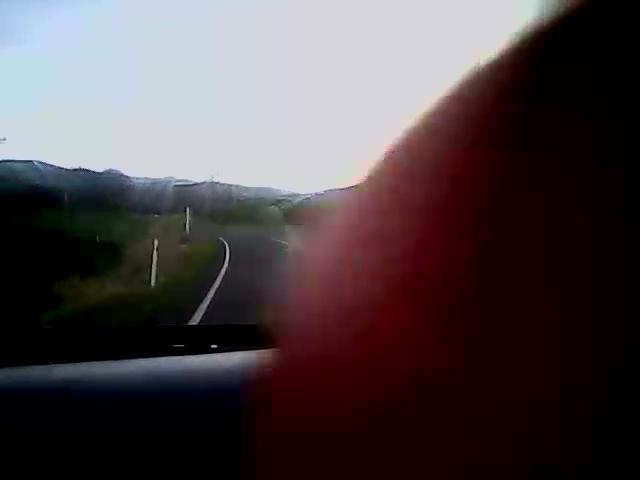The photograph, taken from inside a car, captures a scenic roadway flanked by a grassy landscape with scattered poles and a backdrop of towering, dark mountains under a clear, gradient sky. The image includes parts of the car's interior, such as the gray door frame, dashboard, and black windshield wiper, with the back seat visible. The right side of the photo is partially obstructed by what appears to be someone's thumb, and the overall image is somewhat blurred, adding to the sense of motion and journey. The sunlight illuminates the landscape, creating a bright, daytime scene.